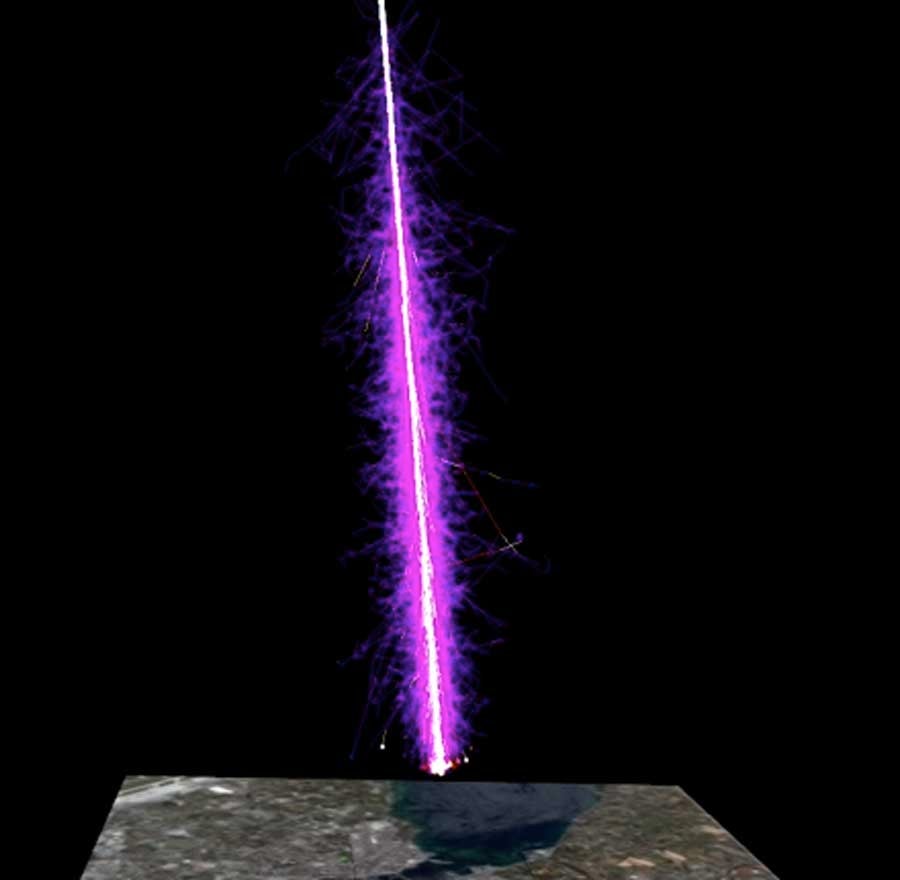The photograph depicts a striking neon pink and purple light streak illuminating a solid black background. The light, resembling a laser ray or molten strike, stretches vertically from the top of the image toward the bottom, terminating just short of a small, concrete or marble table. The light is predominantly white at the core with a vibrant, almost sparkly neon pink aura around it. This mysterious beam creates a stark contrast against the encompassing darkness, evoking a sense of movement and intensity, as if it's shooting upwards or descending from the sky. The table beneath, with its concrete-gray surface and a speck of dark color in the center, adds an intriguing foreground to this enigmatic scene.